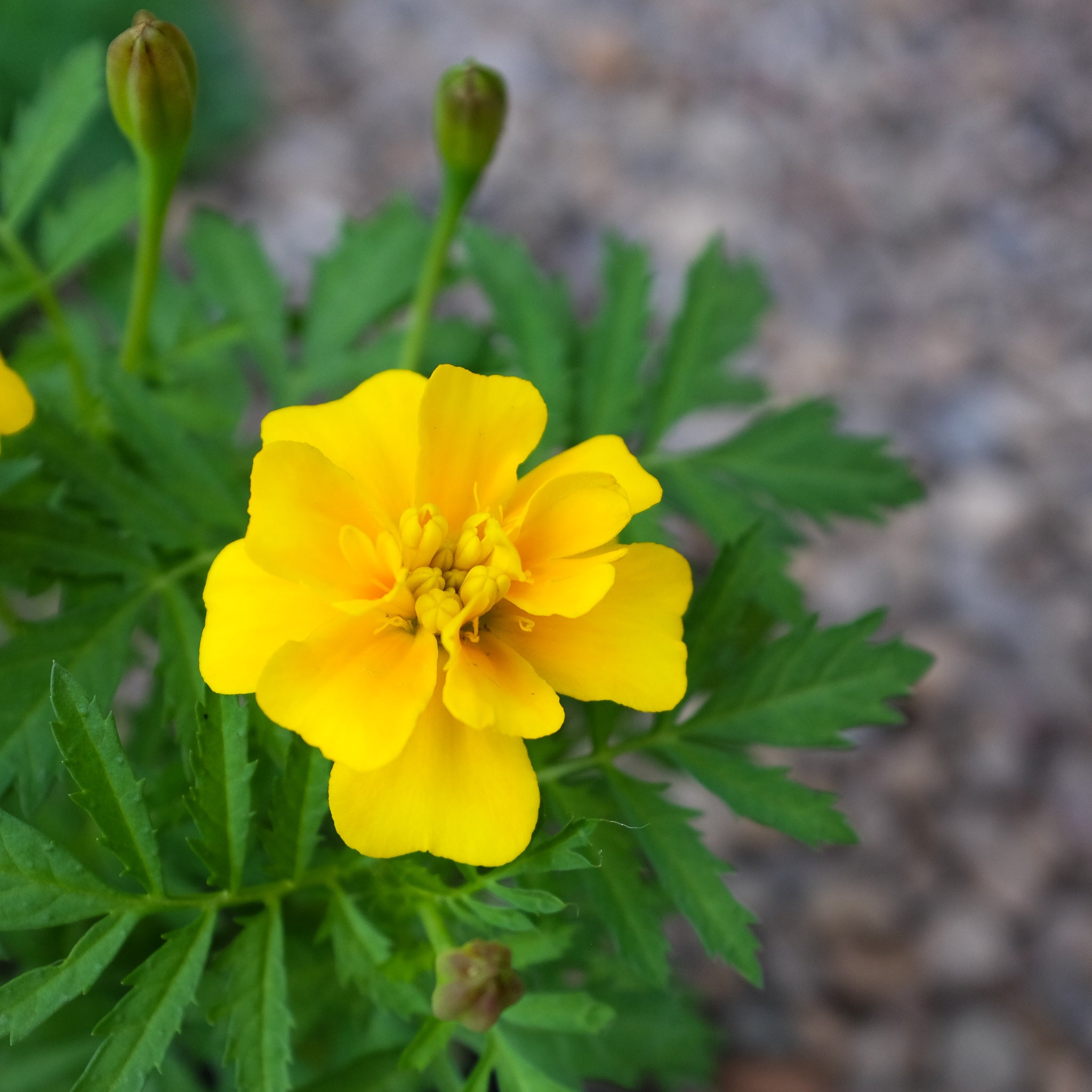This close-up photograph showcases a vivid yellow buttercup flower in full bloom. The flower has two distinct rows of delicate, bright yellow petals—each row featuring five petals. The innermost area of the flower reveals its reproductive parts, including stamens and emerging buds, some of which appear to have petals of their own. The cheerful buttercup is set against a backdrop of bright green leaves that are pointy and jagged-toothed, arranged in small clusters along the stem. The background is a blurry, grayish-brown expanse, suggesting the flower is situated in a natural, possibly hilly environment.